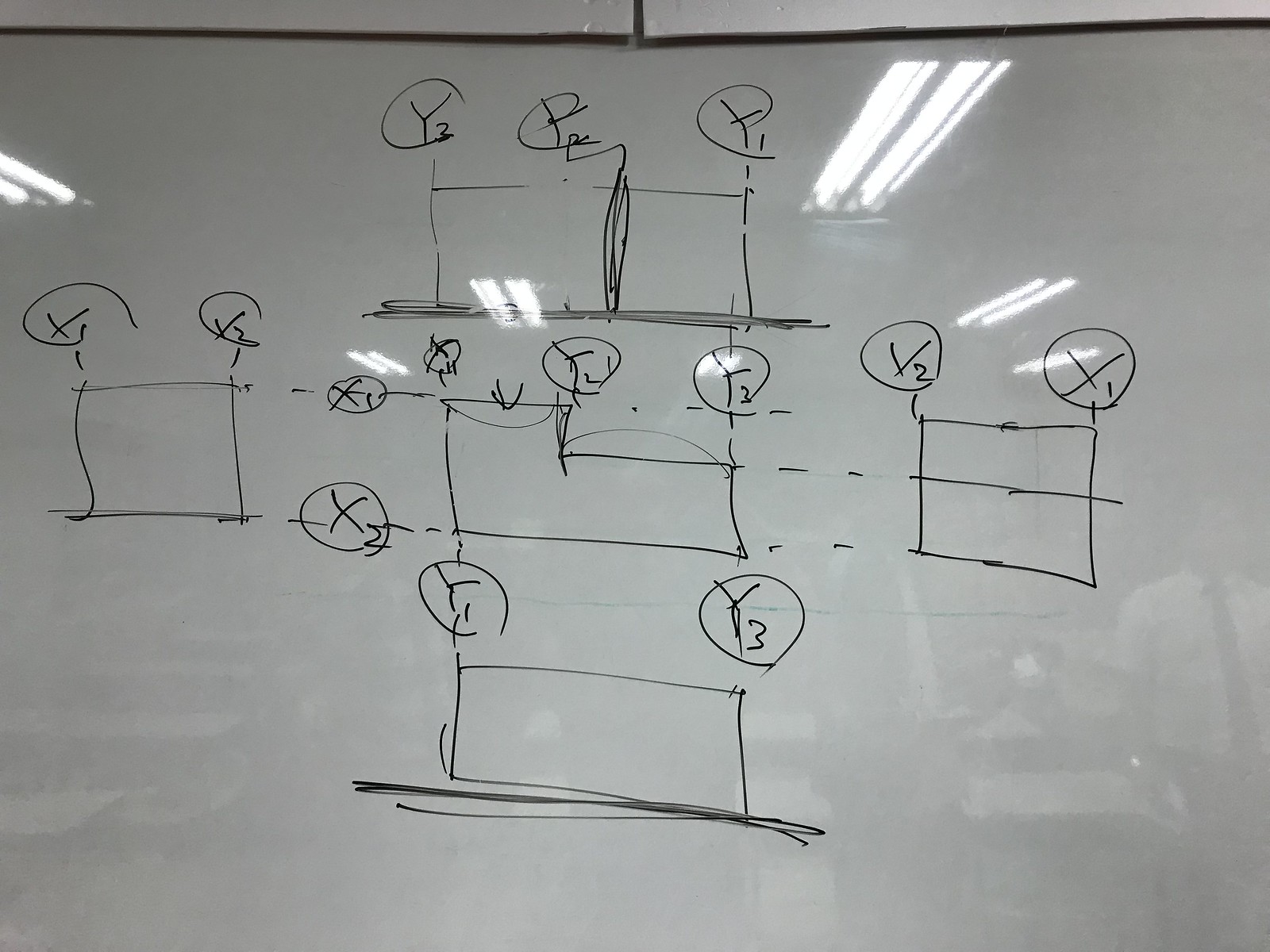The image depicts a whiteboard with a hand-drawn diagram composed of multiple squares, likely related to a geometry lesson. The diagram is somewhat messy and appears to be the work of a math teacher, illustrating the process of solving different segments within the squares. The whiteboard itself has a glossy surface, reflecting overhead lights and even revealing the faint outlines of students who are attentively observing the board. This cluttered, yet instructional display captures a typical classroom setting where complex mathematical concepts are being explored.